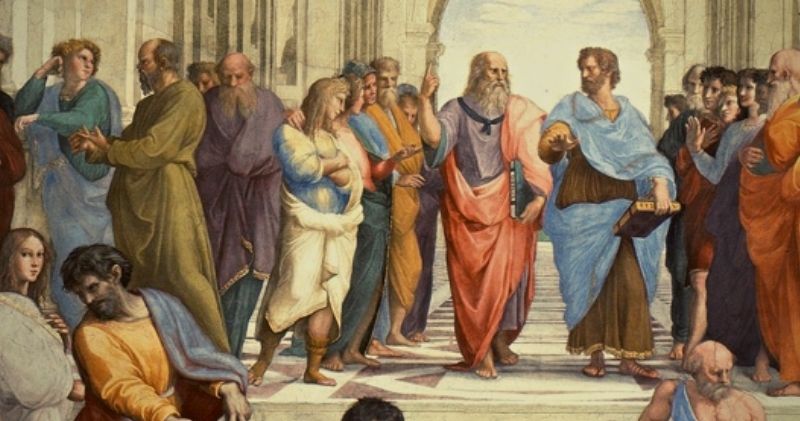The illustration depicts an ancient courtyard scene, possibly from Greek or Roman times, filled with various figures dressed in multicolored robes, ranging from red, blue, orange, white, purple, to green. In the foreground, two men, one older and one younger, walk together under a stone archway. The older man, bald with a large white beard, is attired in a purple shirt with a pinkish-red drape and is barefoot, holding a book while pointing upwards. The younger man, with short brown hair and a short beard, wears brown clothing with a blue drape and a necklace, and might be wearing sandals. He too holds a book and is gesturing animatedly. Surrounding them, groups of people are engaged in various conversations and gestures, with some in the front sitting and conversing amongst themselves. The background shows the courtyard extending into a stone archway, leading outside where clouds are visible in the sky. This bustling scene captures a moment of intellectual discourse and social interaction in an ancient setting.